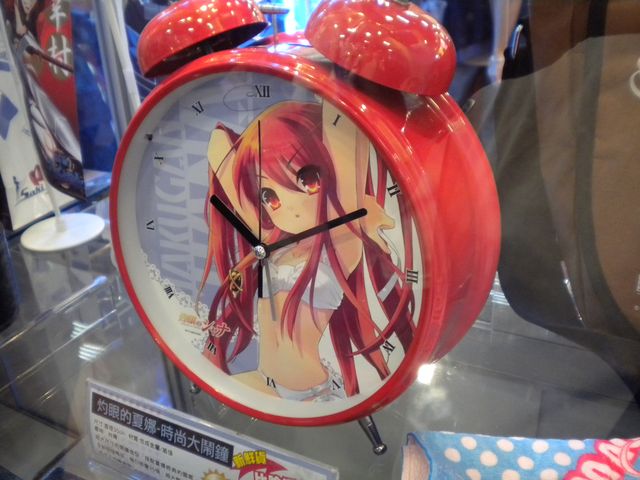This photo appears to have been taken through a display case in a shop, likely an Asian novelty store or located in Asia, given the presence of multiple displays featuring both English and Asian languages. Central to the image is a vintage-style red alarm clock, distinguished by its two bells on top and a small metal hammer that oscillates between them. The clock face features an anime character with large, glowing reddish eyes and long red hair, dressed in a bathing suit. Surrounding the alarm clock are various other products, including a backpack and a blue blanket with white polka dots and red lettering, though the specific details of the lettering are obscured. The background includes additional items and signs with Asian script, enhancing the cultural context of the scene.